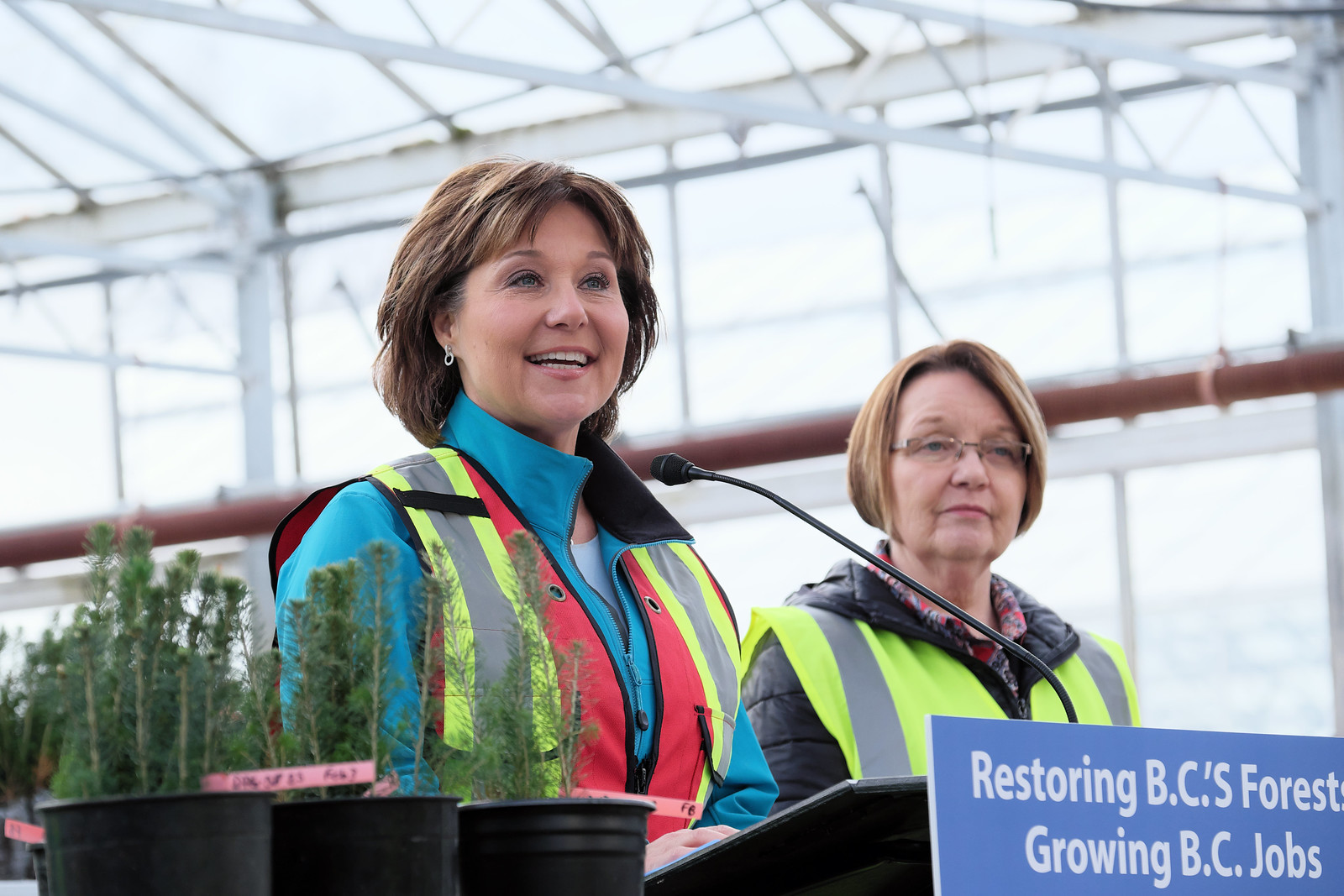In the image, two Caucasian women are standing at a black podium inside a greenhouse characterized by numerous glass windows on both the walls and ceiling, allowing a view of the sky from every angle. The podium features a blue sign with white text that reads "Restoring BC's Forests, Growing BC Jobs," and it is equipped with a black microphone. Both women are dressed in high visibility vests: one with lime green and silver stripes, and the other with additional red detailing. The woman on the left is wearing a light blue zip-up jacket under her vest. She has short blonde hair that reaches her neck. The woman on the right wears her short blonde hair down around her face, sports glasses, and has a black puffer winter jacket under her green and silver safety vest. Surrounding the podium are plastic pots with various herbs and small trees, hinting at the greenhouse's agricultural setting.